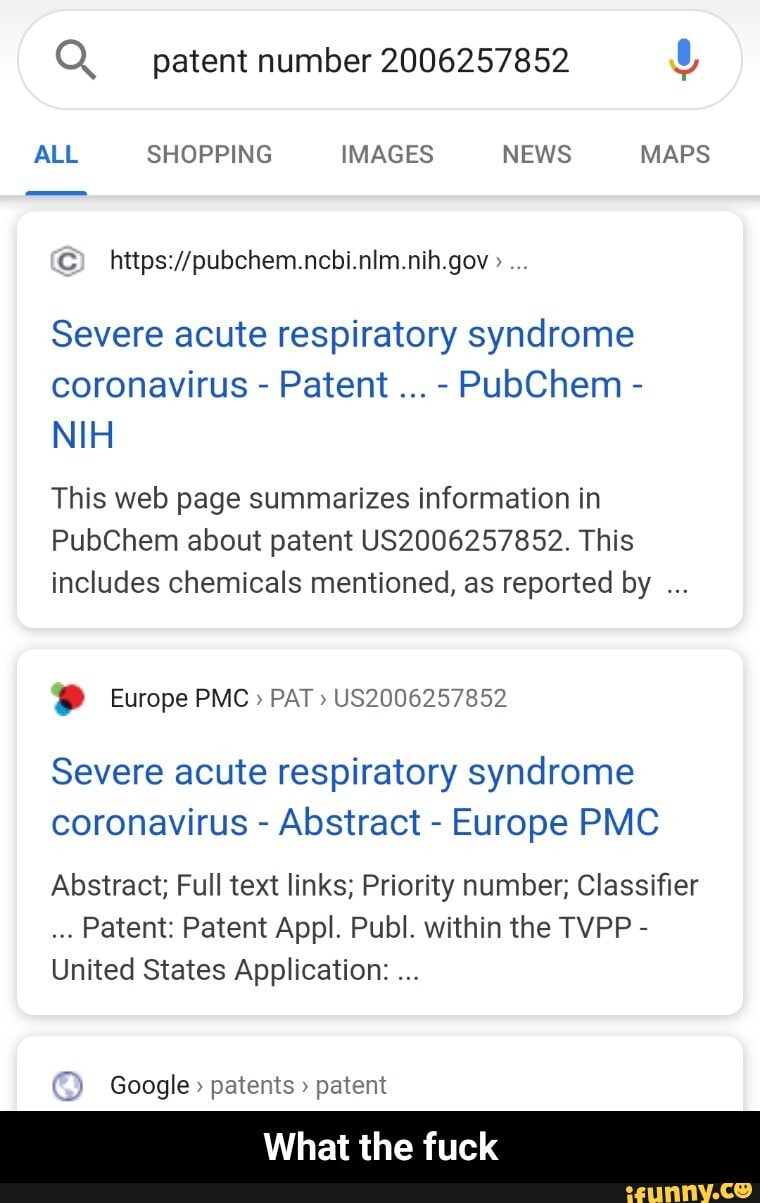Screenshot of a Google search result on a mobile device. The background is grey, with a white search bar in the center. On the left of the search bar is a magnifying glass icon in grey or black. The search query reads "patient number 2006257852," accompanied by a multicolored microphone icon (blue, green, yellow).

Below the search bar, the options for "All," "Shopping," "Images," "News," and "Maps" appear in blue and grey text respectively. The results include two website links: 

1. The first link features a black website address. The blue text reads "Severe acute respiratory syndrome, contagious, coronavirus, patient, PubChem, NIH". Below, in black text: "This webpage uses patient information, PubChem, patient," and the search number. It continues: "This includes chemicals mentioned as reported by..."

2. The second link begins with "Europe PMC" in grey, followed by the search number. Blue text reads "Severe acute respiratory syndrome, coronavirus, abstract, Europe PMC". Below, additional links include "abstract, full text links, priority," and more.

At the bottom, a black bar with white text reads "what the fuck." On the right-hand side of this bar, a red line and grey text indicate "ifunny.co".